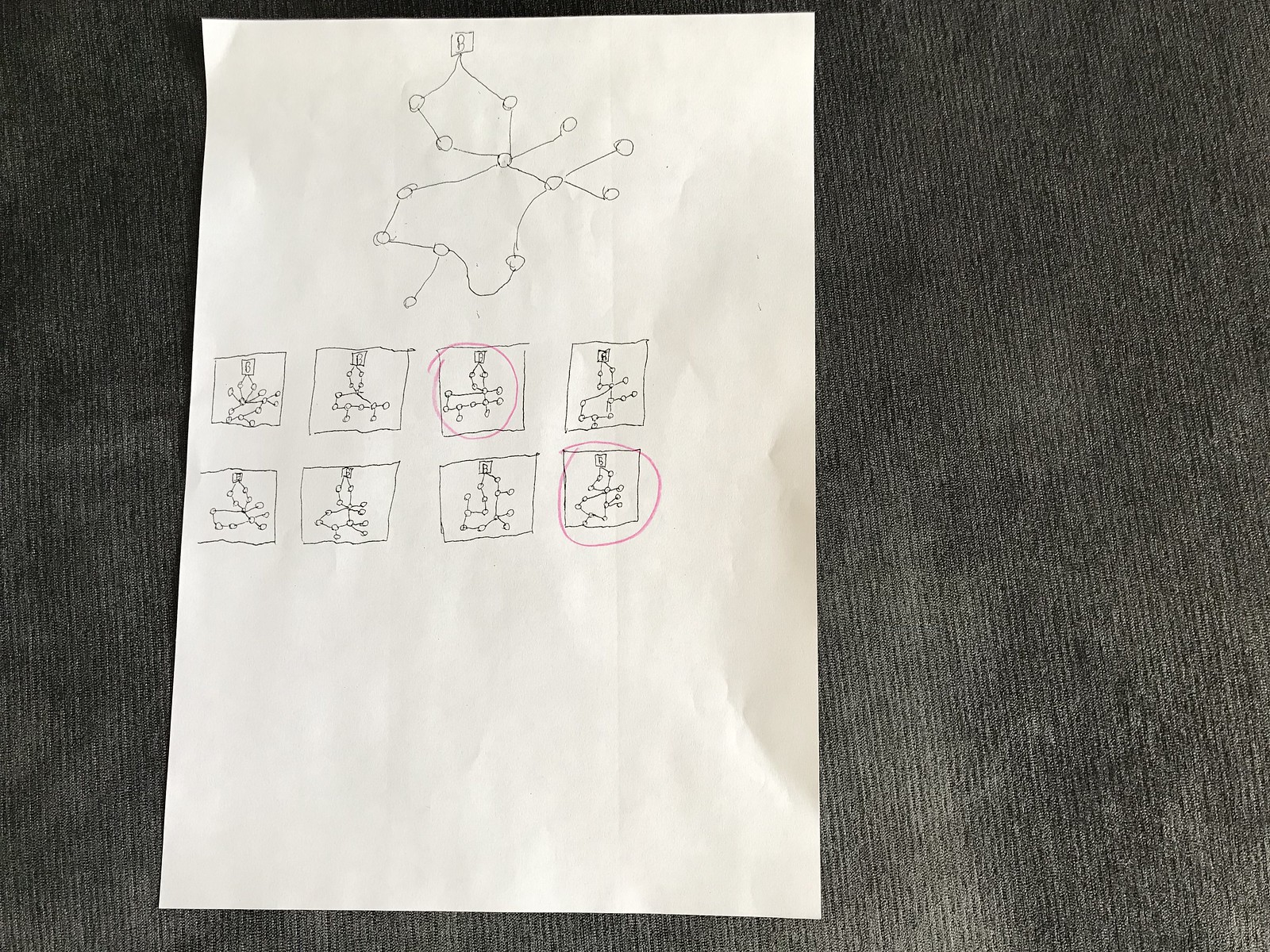This photograph features a slightly curled and wrinkled sheet of unlined white paper, set against a textured black fabric background reminiscent of corduroy. The paper is covered in intricate drawings rendered in black ink or pencil. At the top, a large illustration displays a network of connected lines interspersed with small circles, crowned by a small square containing the letter "B." Below this, the paper is divided into eight smaller illustrations, each neatly enclosed within its own square. These smaller diagrams also consist of various lines and circles, with each bearing a square labeled with the capital letter "B" above it. Notably, a red circle highlights two of these smaller illustrations: the third diagram from the left in the top row and the far-right diagram in the bottom row.